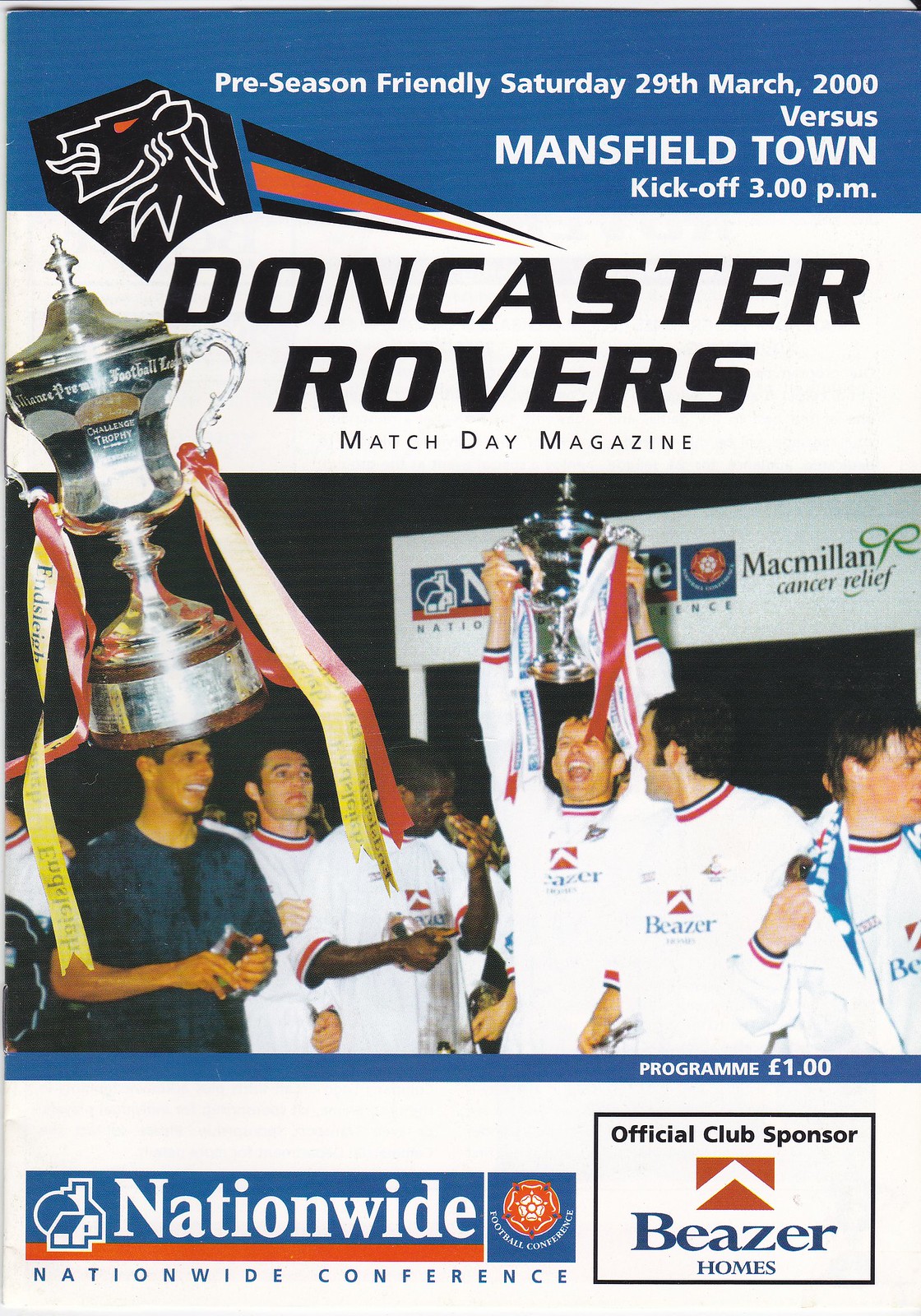The image is a tall, rectangular poster, likely a cover for a football match program or magazine. At the top, a bright blue rectangle features a unique logo on the bottom left: a black shape with a white outline of a lion's face and a red eye. To the right, in white font, it reads: "Preseason Friendly, Saturday, 29th March 2000 versus Mansfield Town, kickoff 3 p.m." 

Below this, in a thick white rectangle, the text "DONCASTER ROVERS" is written in bold, black, all-capital letters, with "Match Day Magazine" underneath in smaller text. 

The center of the poster showcases a wide photograph of a soccer team dressed in white shirts with red and black details, celebrating and holding a large silver trophy adorned with red and yellow ribbons. One player prominently holds the trophy up, smiling broadly. The front of the white shirts features the name "Beezer" in blue.

Towards the bottom, within a blue and orange rectangle, it states "Nationwide Conference" and includes the "Nationwide" logo. Additional text at the very bottom indicates the official club sponsor, "Beezer Homes."

Overall, the poster is rich in detail, combining elements of event information, team pride, and sponsorship recognition.